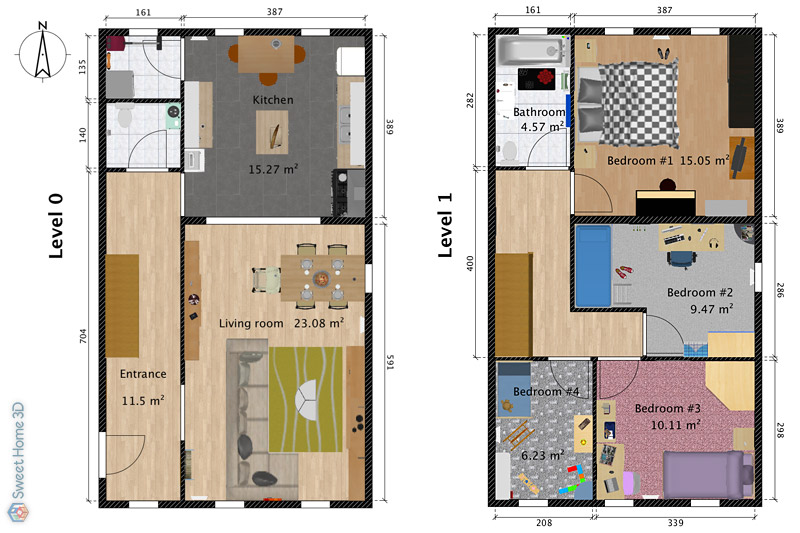This image shows a detailed blueprint layout of a two-level home, clearly marked as Level 0 and Level 1. The blueprint appears in color and includes all measurements and the square footage of each room, with an arrow in the top corner indicating the north direction. The diagram seems to be from a service called Sweet Home 3D, as indicated by its logo on the side.

Level 0, depicted on the left, includes the entrance at the bottom left, leading into a hallway that connects the living room on the bottom right, the kitchen at the top right, and a bathroom at the top left. The kitchen also connects to what appears to be a small closet or laundry room. The positions of all doors and their swing directions are specified.

Level 1, shown on the right, consists of four bedrooms: a larger bedroom at the top right, two average-sized bedrooms at the bottom left and bottom right, and a smaller bedroom near the top left. This floor also includes a bathroom at the top left and a connecting hallway. All closets and door placements are shown in detail. The room sizes are numerically labeled, providing a comprehensive overview of the space available in each area.